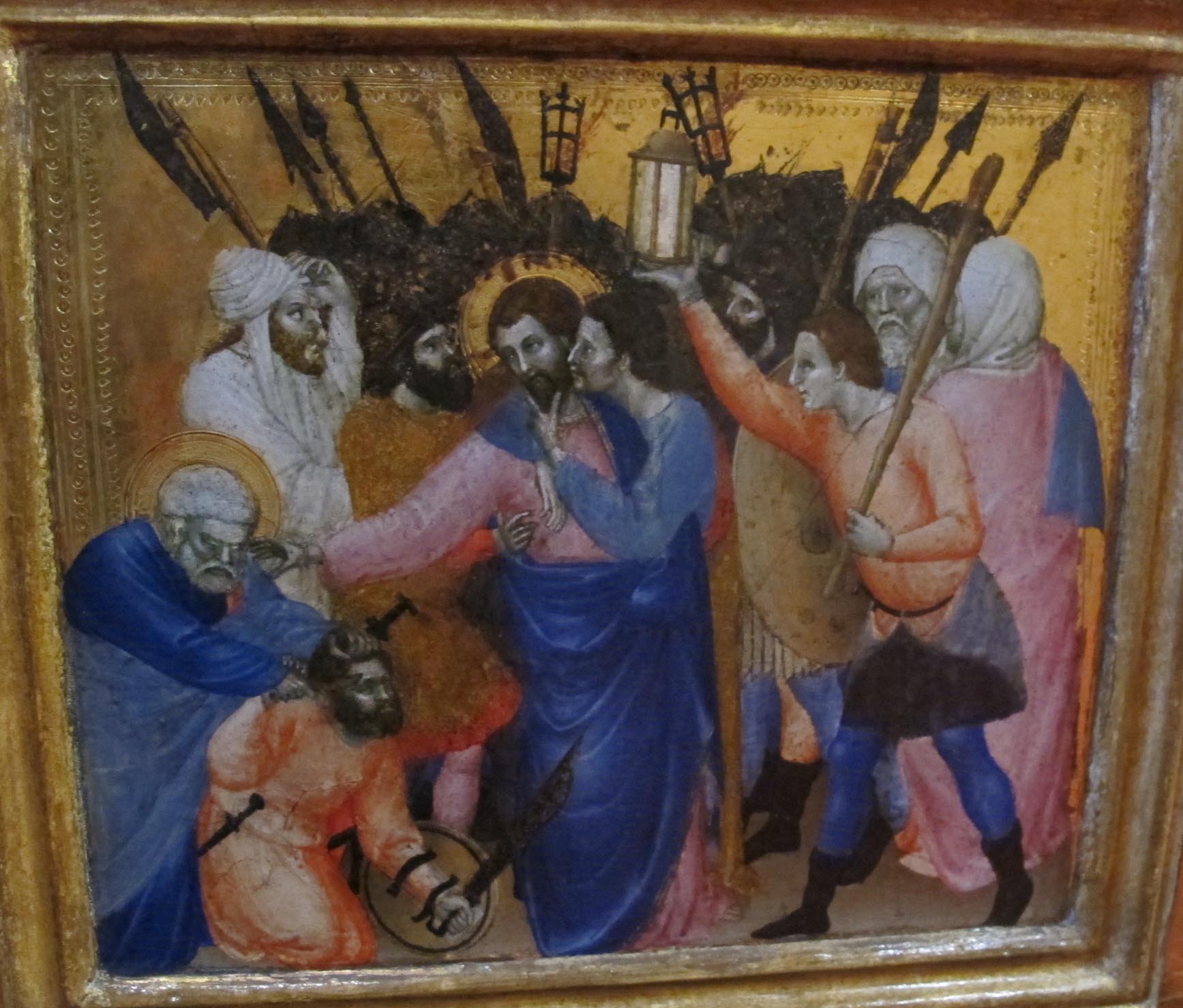The medieval-style painting, framed with a gold border and a yellowish backdrop, showcases a deeply religious scene centered around a Christ-like figure. This central figure, dressed in traditional robes, appears to be beseeching or blessing someone to cease an act of violence. Surrounding the Christ-like figure are nine armed men, some wielding swords, bows, and lanterns. To the right, a man in a peach-colored shirt holds a lantern and a stick, while on the lower left, another man in a similar peach robe grasps a shield and sword. A dramatic interaction unfolds at the bottom, where a man is held down by another who grips his hair and holds a knife to his head, representing a moment of intense conflict. This scene is a vivid tableau of confrontation and compassion, embodying the essence of its religious and historical implications.